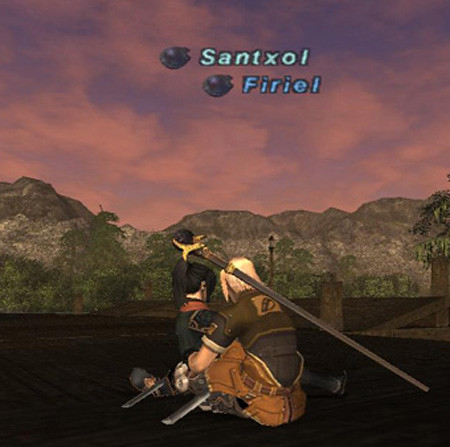The image appears to be a computer-generated scene, resembling the graphics of a video game. It features two characters, a man and a woman, seated on a wooden platform. Both individuals are facing away from the camera, with the man positioned closer to the center of the frame and the woman sitting slightly in front of him. The man's back is adorned with a long sword, while the woman has black hair styled in a ponytail. In the background, a wooden walkway or bridge extends into the distance, leading towards a rugged mountain landscape under a purplish-red sky. The overall scene conveys a sense of adventure and mystery, enhanced by the vivid and fantastical environment.